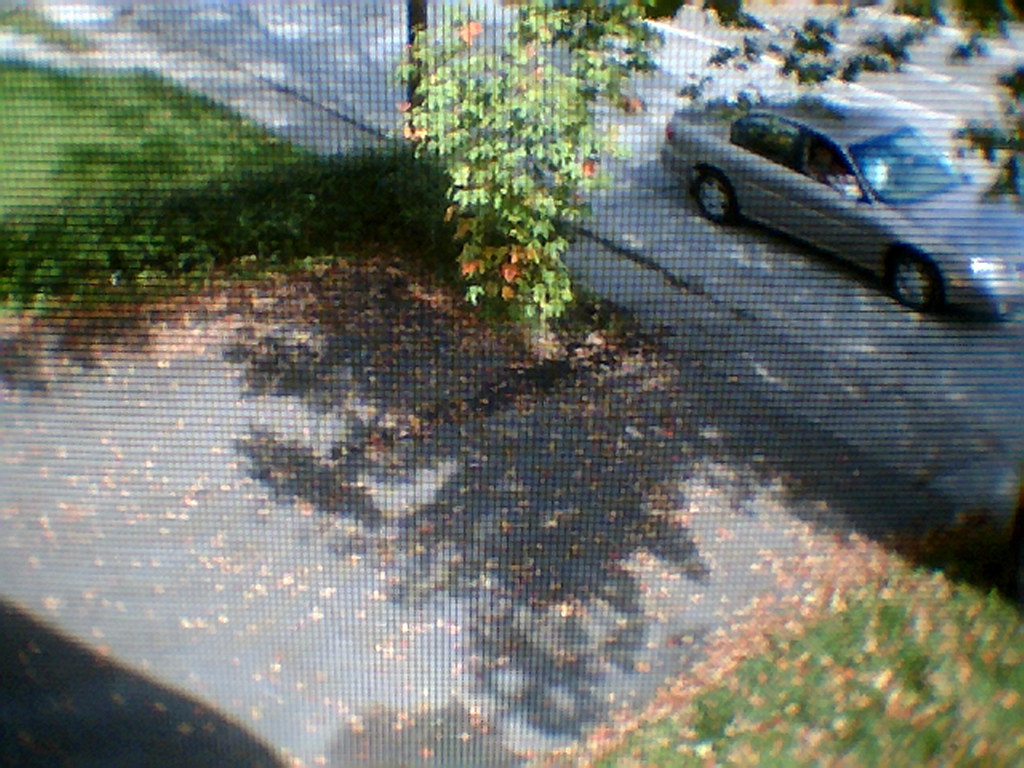Through the mesh of a window screen, an asphalt driveway comes into view, its dark surface contrasting against the green grass framing its edges. Scattered dried leaves line the perimeter where the driveway meets the lawn, adding a touch of autumnal decay to the scene. Dominating the composition is a large tree, its expansive canopy casting shadows over the driveway, the adjoining sidewalk, and a car parked by the curb. The interplay of light and shadow, combined with the natural elements, creates a serene suburban tableau.